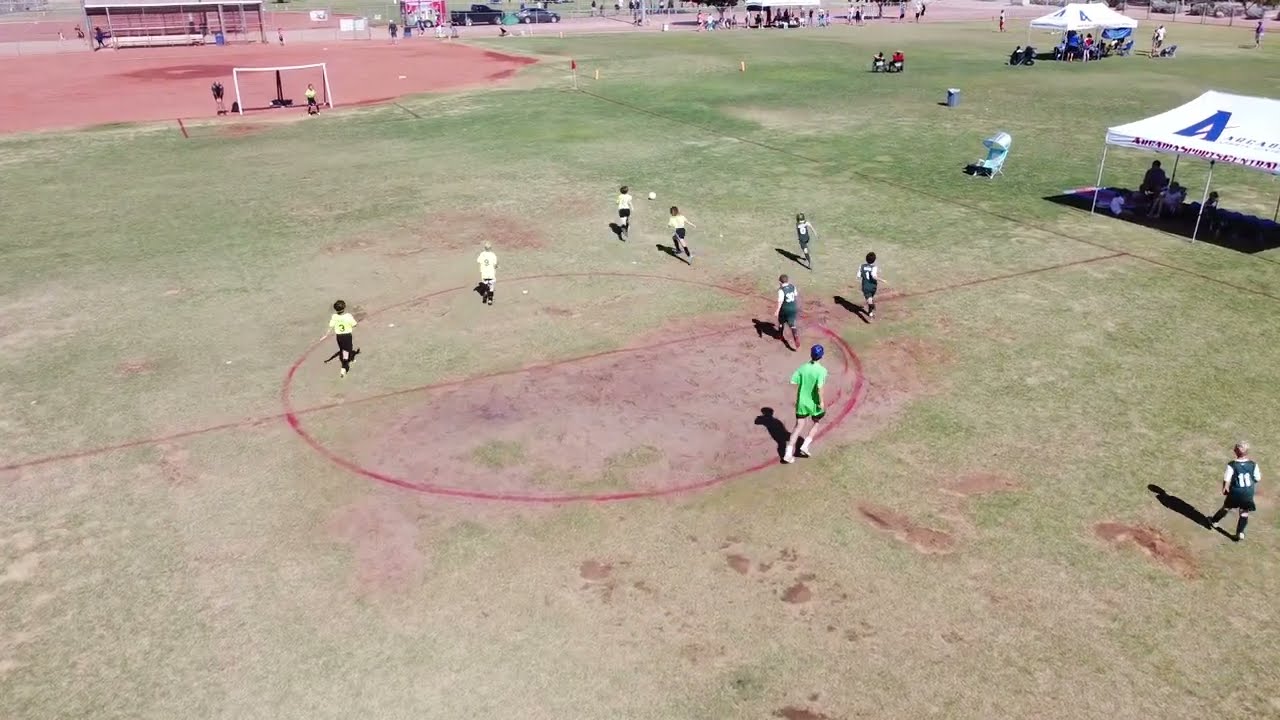This photograph, captured from a higher vantage point, shows an energetic soccer match on a large athletic field. The scene is bustling with young players in various uniforms; there are four players in yellow jerseys, four in darker blue jerseys with white sleeves, and a player in a bright green jersey who appears to be the referee. All players are wearing black shorts, tall black socks, and white shoes. A yellow-jerseyed player, facing away from the camera, is sprinting towards the soccer ball, which is positioned near the top of the photo. 

The field itself is marked with red lines, including a prominent center line and a large red circle indicating the middle for scrimmage. To the right of the soccer field, a group of spectators sits in the shade beneath white tent canopies, and a person in a lawn chair can be seen closer to the action, observing intently. 

In the background, beyond the soccer field, is a baseball or softball stadium, identifiable by a dugout, home plate, and dirt infield. Farther back, another soccer net is visible, possibly indicating an adjacent field. A stroller is also noticeable among the onlookers. The overall scene is vibrant and active, highlighting both the excitement on the field and the engagement of the spectators.